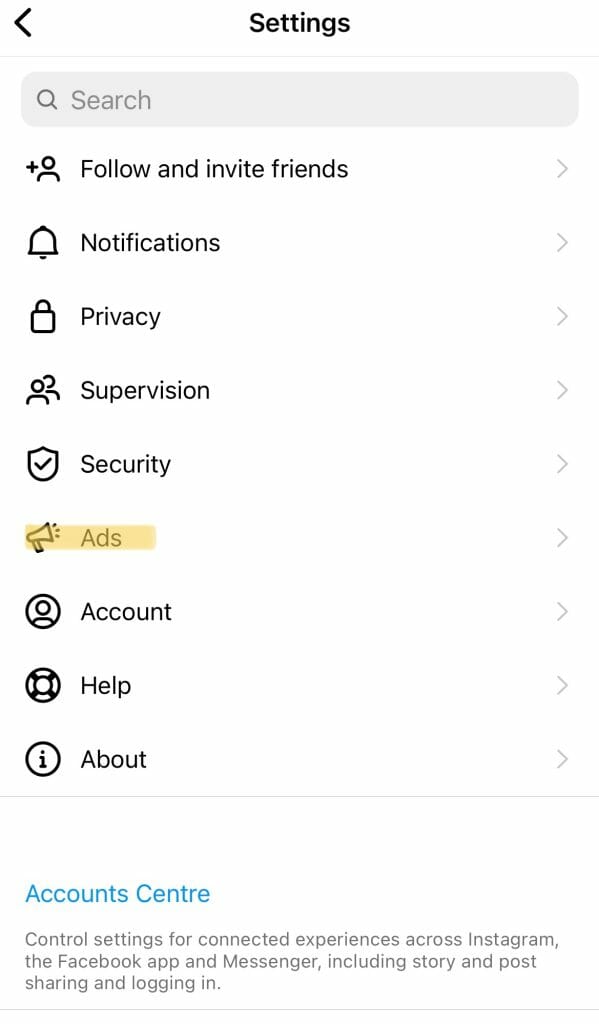The image depicts a vertical mobile screenshot of a settings menu. The background is white, and at the very top, the word "Settings" is written in black, accompanied by a left-facing arrow on the left-hand side. A thin gray horizontal line spans from left to right directly beneath the title.

Below this line, there is a gray search bar with a search icon on the left and the word "Search" inside. The menu consists of several options, each accompanied by a small gray arrow on the right. The options listed from top to bottom are:

1. **Follow and Invite Friends**: Icon of a plus and a stick person.
2. **Notifications**: Icon of a bell.
3. **Privacy**: Icon of a lock.
4. **Supervision**: Icon of two people.
5. **Security**: Icon of a shield with a check mark.
6. **Ads**: Icon of a megaphone, with the word highlighted in yellow.
7. **Account**: Icon of a circle with a person inside.
8. **Help**: Icon of a life preserver.
9. **About**: Icon of a circle with an "i."

Below these options, "Account Centre" is written in blue, with the British spelling "C-E-N-T-R-E." Underneath this, gray text explains the feature: "Control settings for connected experiences across Instagram, the Facebook app, and Messenger, including story and post sharing and logging in."